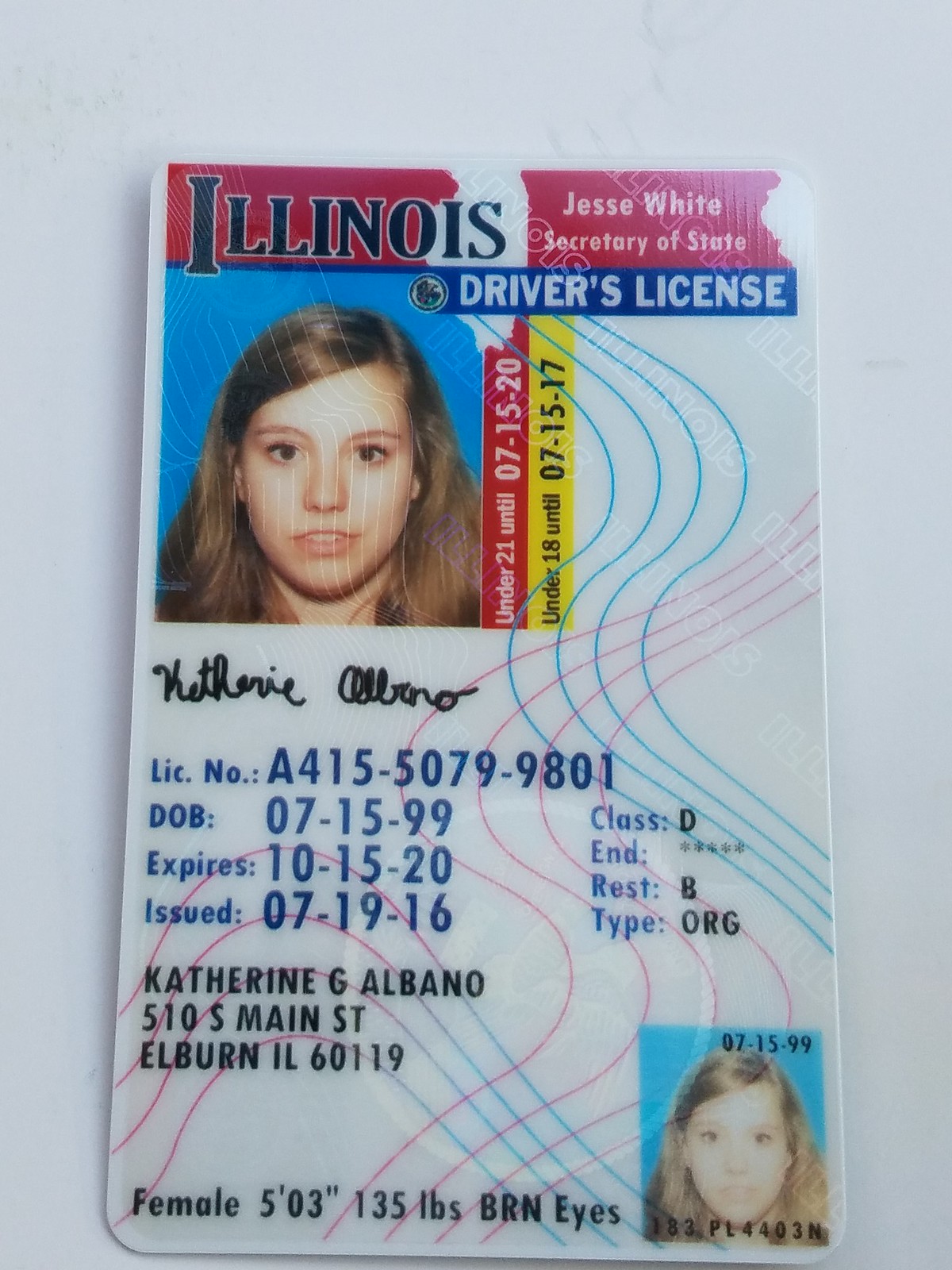This is a color photograph, close-up, of an Illinois driver's license belonging to Catherine G. Albano. At the top, it reads "Illinois, Jesse White, Secretary of State, Driver's License." On the top left, against a blue background, is a photo of a young woman with blonde hair parted on the side. Next to this photo, it states "Under 21 Until 07/15/20" and "Under 18 Until 07/15/17," with her signature below the photograph. The license includes the number A41550799801, her date of birth as 07/15/1999, the issue date of 07/19/16, and expiry on 10/15/20. 

Catherine G. Albano's details are listed as follows: address at 510 South Main Street, Elburn, IL 60119, designated female, 5'3" tall, weighing 135 lbs, with brown eyes. The license is a Class D type, specification 'Rest B.' At the bottom right corner, there is another photo of her.